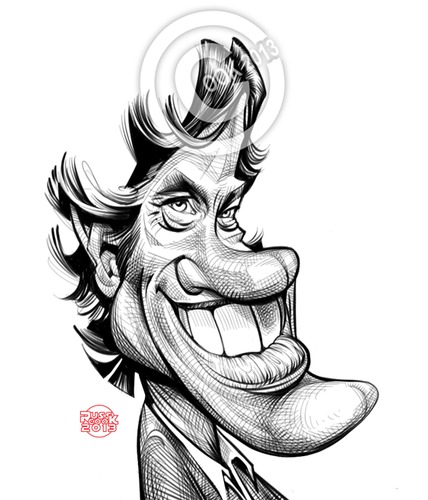This detailed black-and-white caricature drawing, likely created with a pen or very fine pencil, features a highly exaggerated male figure. The man's face is depicted with an oversized chin that juts prominently downward and to the right, an open mouth displaying large upper front teeth, and a protruding nose that extends over the mouth. His forehead tapers to a near point, covered in scraggly dark hair that curls at the ends. Tiny, narrowed eyes sit above a prominent bridge of the nose, and a small ear is tucked behind the scraggly hair. He wears a suit and a white dress shirt with a collar, though the drawing ends before the full upper body is shown. A red circular stamp behind his neck bears the words "Russ Koch 2013." Additionally, at the top of the drawing, there are three gray-outlined white circles with the inscription "00K 2013" integrated into them, possibly serving as the artist's creative watermark or signature. The caricature captures the essence of exaggerated features with whimsical curves, emphasizing the humor and skill involved in such artwork.